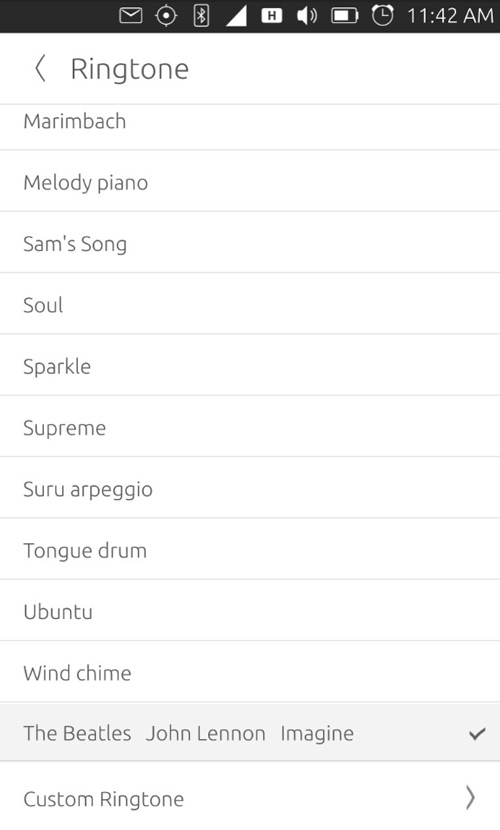The image showcases a cell phone screen where users can select their ringtone. The screen predominantly features a clean, white background. At the top, there is a slim black bar displaying several icons: an email alert, a target symbol (its function is unclear), Bluetooth connectivity, cell signal strength, an "H" likely indicating a connected app, the volume control, battery life, an alarm icon, and the current time, which is 11:42 AM.

Below this, the expansive white space, taking up about 98% of the screen's area, features grey text with various options. At the topmost, there's a back arrow allowing users to return to the settings menu. The title "Ringtone" is prominently displayed.

Listed beneath are various ringtone options: Marimba, Melody Piano, Sam Song, Soul, Sparkle, Supreme, Suru, Arpeggio, Tongue Drum, Ubuntu, Wind Chime, The Beatles, John Lennon, Imagine, and a customizable ringtone option indicated by a right arrow that likely opens a drop-down menu for more options. The currently selected ringtone is John Lennon's "Imagine," which is marked with a check and highlighted in a peach color.